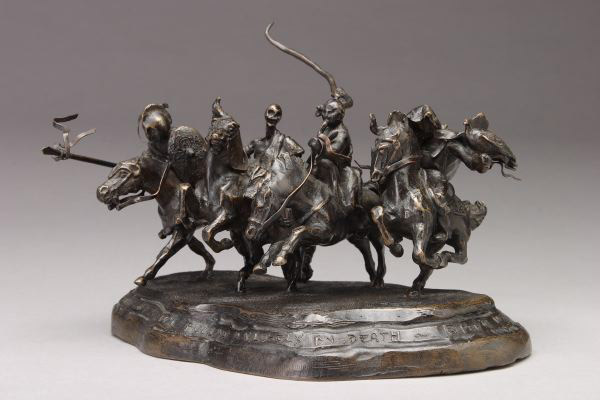The image showcases a captivating bronze statue with a greenish-brown patina, featuring four muscular men in intense combat. The statue, positioned on a plain white surface, depicts the men riding rearing horses, each horse dynamically poised on its hind legs. The base of the sculpture is round with a wavy design and inscribed with text, though "death" is the only discernible word.

Each warrior is depicted in varying action poses, some turning towards the viewer and others away, enhancing the impression of a chaotic battle. The riders are armed with unique and unfamiliar weapons, including a long shaft with curved blades and a five to six feet long curved blade, adding to the drama of the scene. One central figure, adorned in armor, holds a curved horn-like object, while another figure, notable for its skeletal head, has exposed shoulders with armor.

Their faces are contorted in grimaces, suggesting intense effort and struggle. Notably, all the warriors except the skeletal figure are helmeted, adding to the sense of a fierce and tumultuous engagement captured in this detailed and artistic sculpture.